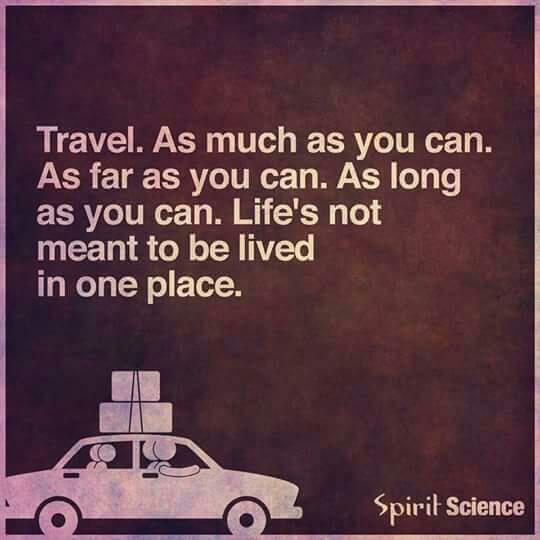The image presents a motivational graphic with a dark brown, reddish-tinted background that has a slightly dated appearance. The centerpiece of the graphic features a simplistic, one-dimensional white illustration of a four-door car, with round-headed, iconic figures representing a family of four inside. The car is depicted with two pieces of luggage or packages tied securely to the roof. Above this illustration, a light cream-colored text reads: "Travel as much as you can, as far as you can, as long as you can. Life's not meant to be lived in one place." The words "spirit science" appear below the image to the right. The overall color scheme blends varying shades of brown with the white text and illustration, creating a harmonious yet motivating visual.